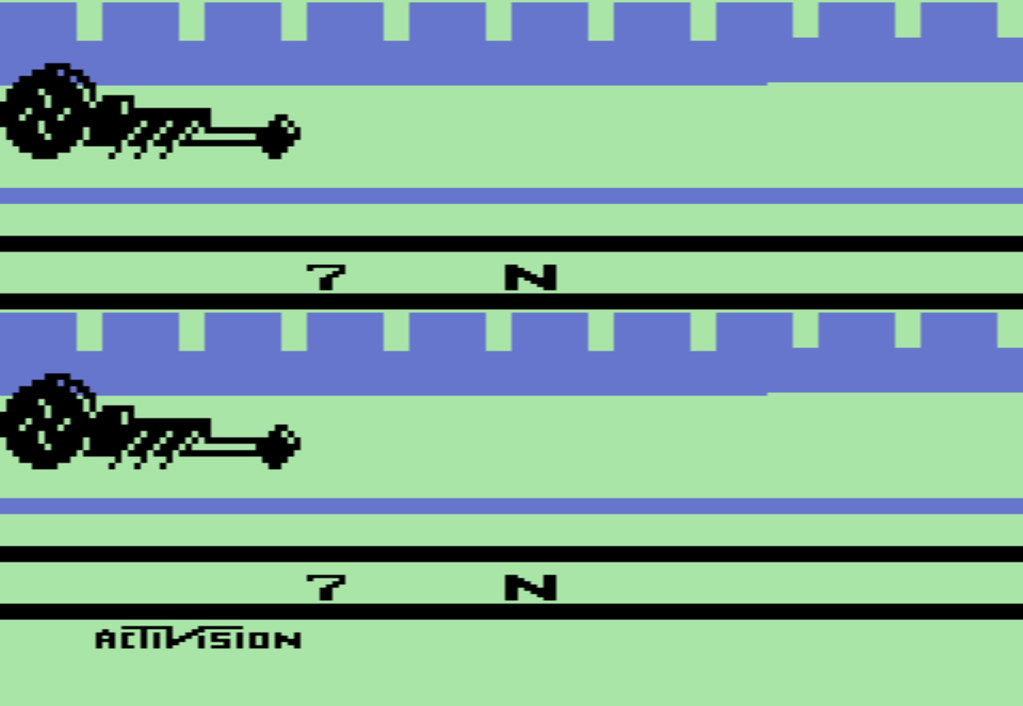In this image, we have a screenshot from the classic Atari video game, Dragster. The scene depicts two players about to race on a green track. The upper half of the screen shows one player's track, while the lower half shows the other player's track. The background features simplistic blue buildings, reflective of the limited graphical capabilities of the era. Each player controls a black dragster, with numerical indicators displaying their current gear status. Both dragsters are presently in neutral gear, gearing up for the race. The game requires players to skillfully manage acceleration to avoid engine explosions, a common hazard in this high-stakes drag racing game.